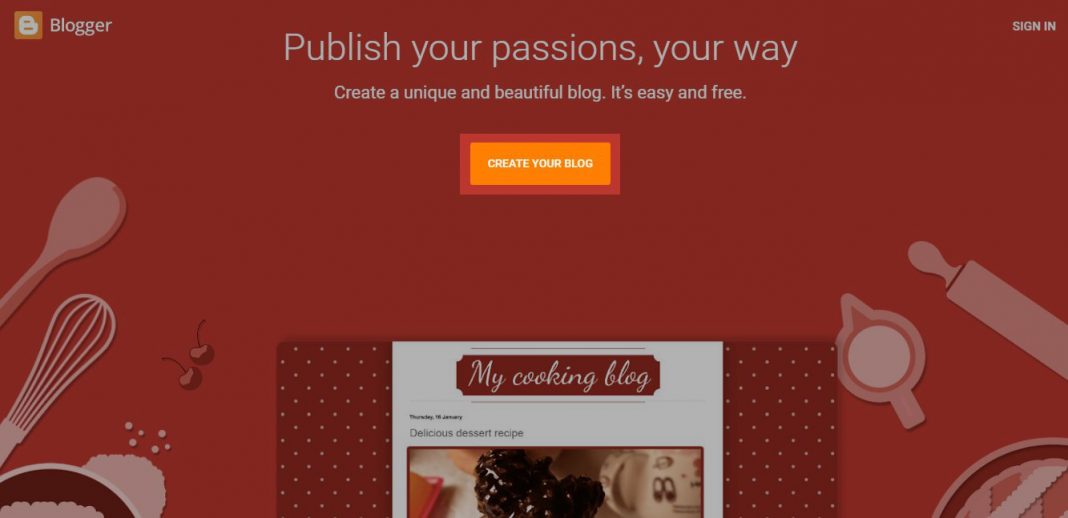This screenshot captures the user interface of a blogging platform. In the upper left-hand corner, the word "Blogger" is prominently displayed, while the upper right-hand corner features a "Sign In" button. At the top center, the text encourages users to "Publish your passions, your way. Create a unique and beautiful blog. It's easy and free." Below this motivational header is a call-to-action button with a red outline, orange center, and white text, reading "Create Your Blog."

Further down, the image features a segment titled "My Cooking Blog" with a timestamp that appears to indicate a Thursday in January, although the exact date is ambiguous. The blog post is titled "Delicious Dessert Recipe," and a partial image of what seems to be a chocolate dessert is visible. The website's background is dark red, adorned with kitchen-themed illustrations. On the left side, there are graphics of a spoon, a whisk, a bowl, some powder, and two stemmed cherries. On the right side, illustrations include a rolling pin, the top of a measuring cup, and the top of a pie.